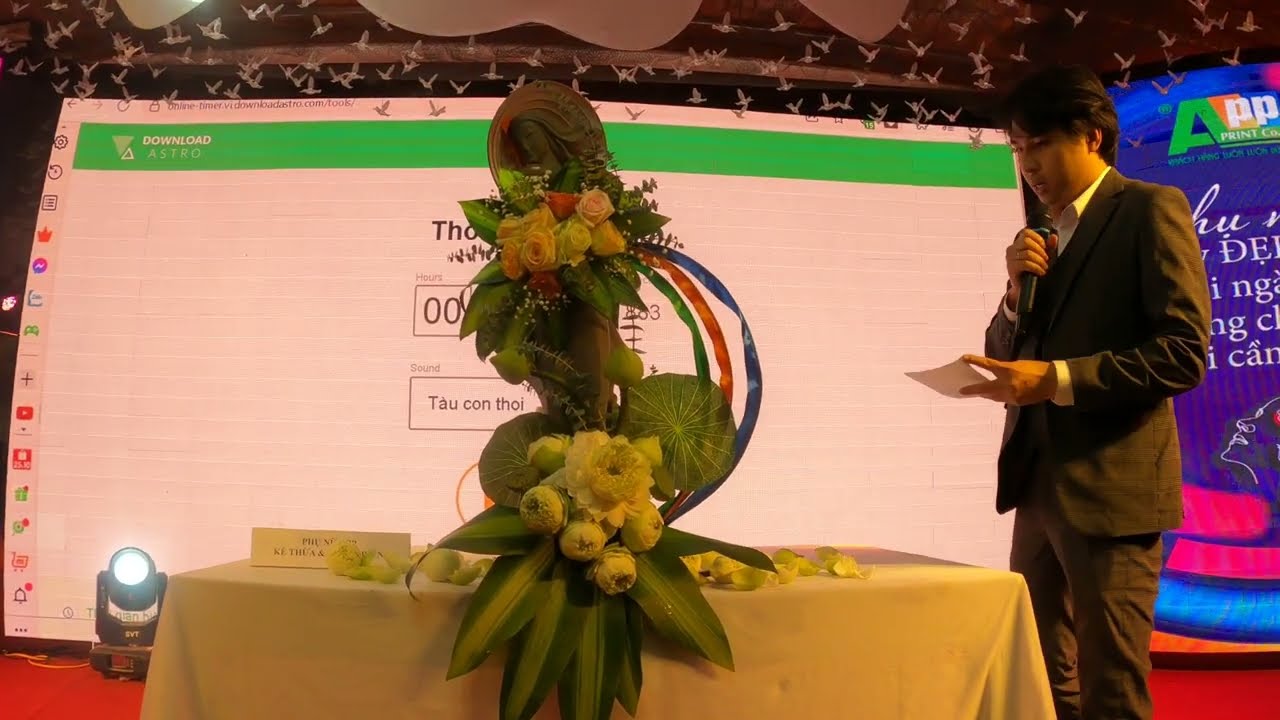The image captures a man standing on a stage, dressed in a white shirt under a black suit, with short dark hair. He is holding a microphone in his right hand while his left hand holds a white paper, with two fingers visible. His mouth is open, showing part of his teeth, as he looks down and talks towards an elaborate plant arrangement placed on a table in the center. The table is draped with a white tablecloth. The plant arrangement comprises green leaves, yellow and red flowers, and appears to include a statue resembling the Virgin Mary adorned with floral decorations. To the left side of the image, there's lighting equipment visible. Behind the table and plant arrangement, a large screen displays a white background with a green bar featuring some text in a foreign language and the words "Download Astro" in the top left corner. Additionally, cute, whimsical paper birds hang from the ceiling, contributing to the festive atmosphere of the event.